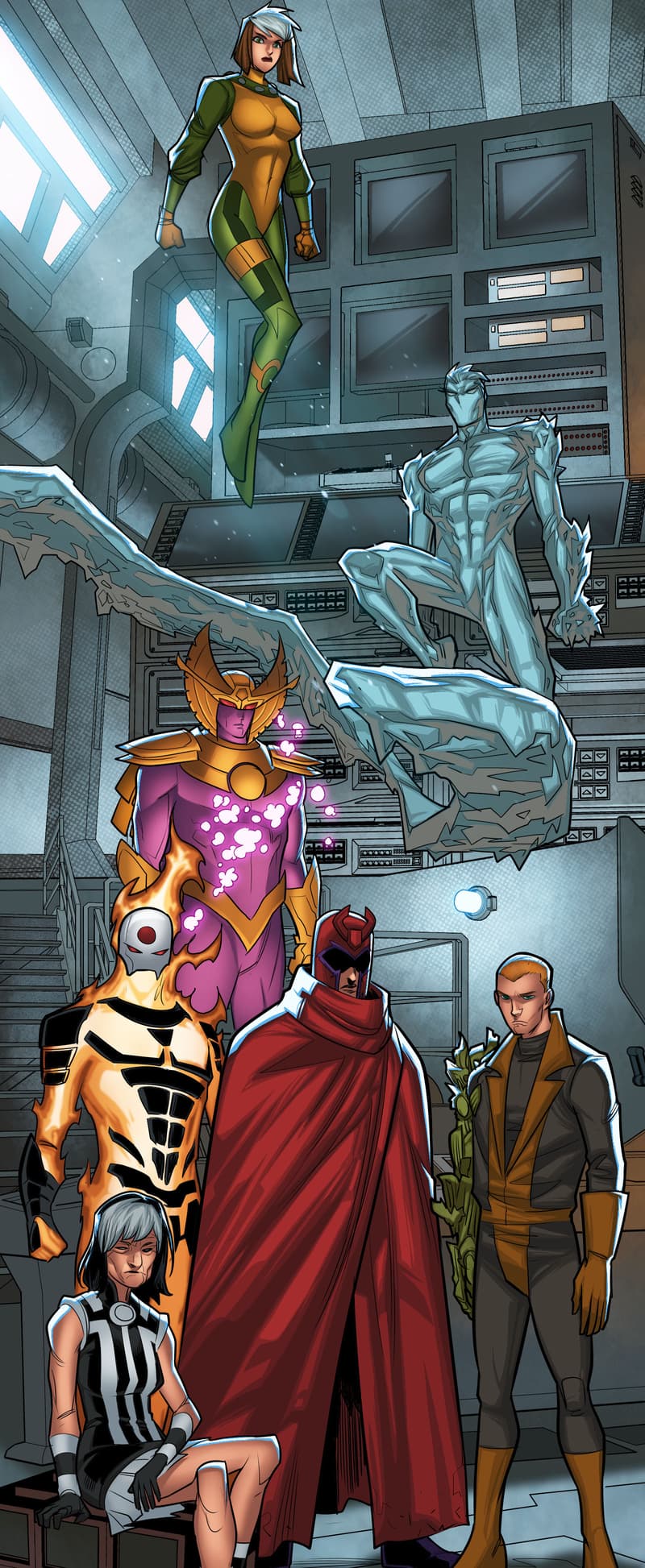This detailed color illustration, inspired by Marvel's Age of Apocalypse, features a diverse array of characters in a portrait-oriented, comic book style scene set against an industrial gray backdrop filled with computers and monitors. At the top left floats a female character adorned in a gold chest plate, long-sleeved green top, green tights, and a matching cap over her brown hair. To her right, an Iceman figure emerges from a winding ice path, devoid of facial features with icy shapes accentuating his shoulders and wrists. Dominating the bottom center stands a red-caped figure: clad entirely in red with a face mask and devil horns, his flowing cape wrapped around his neck. To his right, a young man in a brown tunic with a green arm and a gloved hand contrasts sharply with his surroundings. Above the caped figure, a regal character showcases gold wings on either side of its head, donned in a purple outfit. Positioned slightly below and to the left, a gleaming gold figure with black plates spots a white skull cap and flames crowning its head. At the bottom left, another youthful figure, possibly female, wears a gray and black striped tunic top with a matching skirt, complemented by long gray hair. The detailed artwork combines elements of heroism and enigma, unified in a futuristic, tech-laden environment.